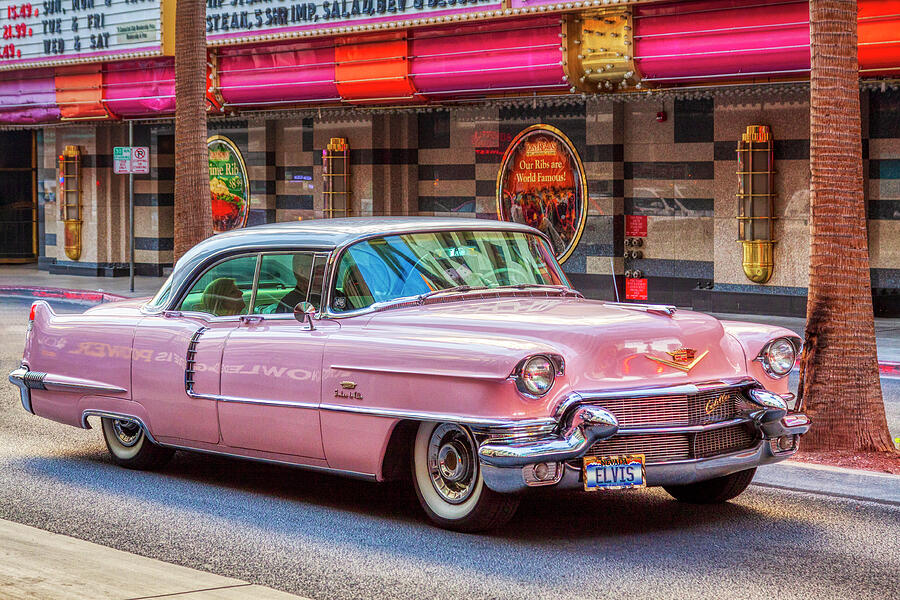In front of a vibrant granite stone building, which features a mix of pinkish, black, and burgundy blocks arranged without any particular pattern, a long-bodied classic Cadillac from the 1950s is parked next to the curb. This vintage car, painted in a striking baby pink color, boasts gleaming chrome bumpers, trim, and white sidewall tires, indicative of meticulous restoration. The Cadillac emblem is proudly displayed on the front hood, and the Nevada license plate reads "Elvis." The building, likely a theater given its brightly colored lights and prominent billboard announcing shows, adds to the scene's lively atmosphere. Palm trees line the curb, enhancing the classic Las Vegas strip aesthetic, complete with neon signs and restaurants in the background.